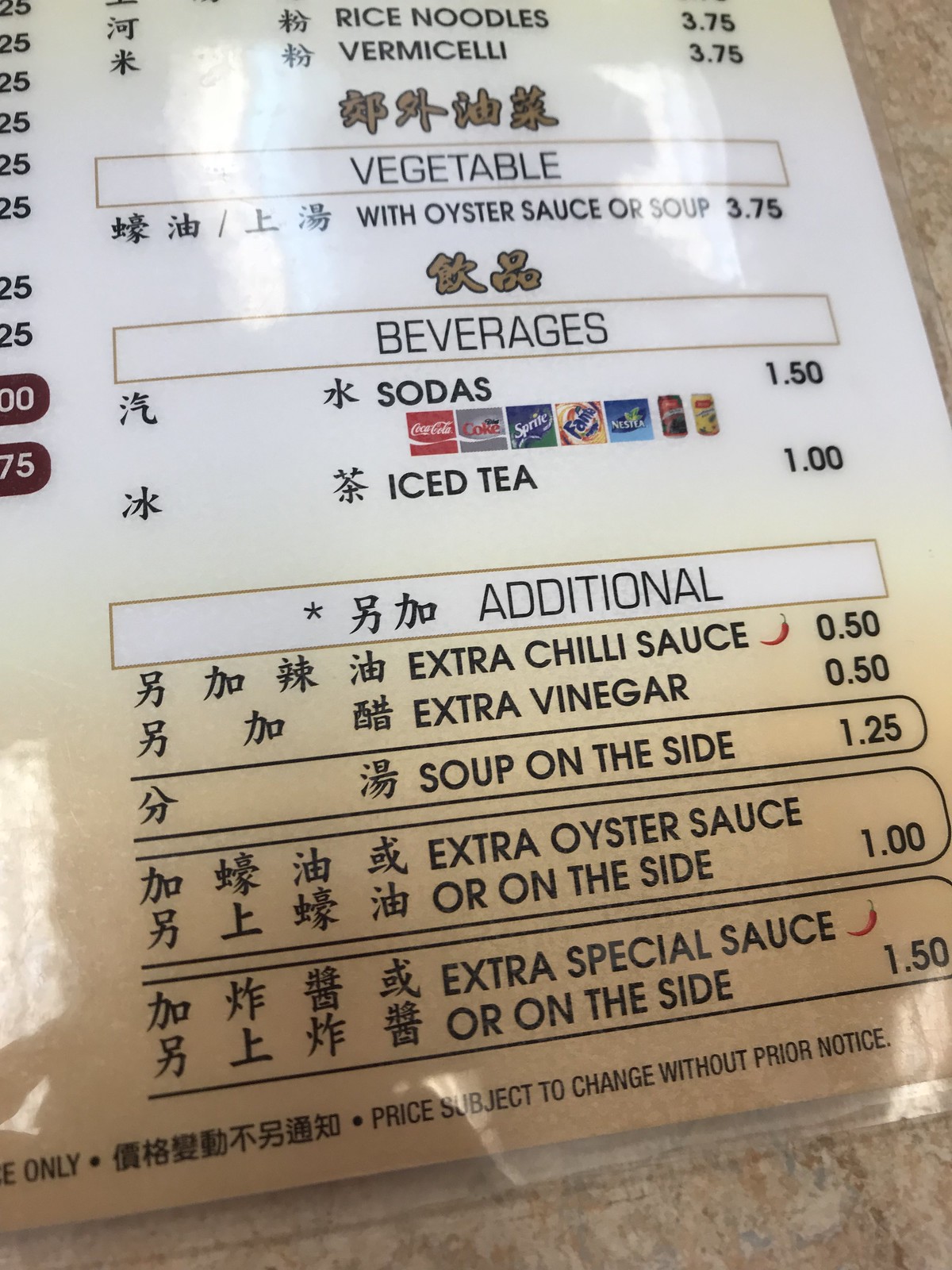This menu, encased in a white plastic sleeve, features a variety of Asian food options presented in both an Asian language and English. The excerpt shown highlights several sections. 

Under the "Vegetable" category, which may include dishes such as vegetables with oyster sauce or vegetable soup, a dish is priced at $3.75. Also pictured are offerings listed under "Rice Noodles and Vermicelli."

The beverages available are sodas and iced tea, as noted in the "Beverages" section.

Additionally, there is a section titled "Additional," which allows for various add-ons such as extra chili sauce, extra vinegar, soup on the side, oyster sauce, and extra special sauce, with all options clearly presented in both languages.

A disclaimer at the bottom notes that prices are subject to change without prior notice.